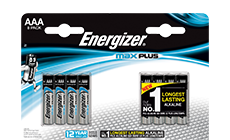In this image, set against a plain white background, we see a detailed screenshot of a package of Energizer batteries. The package is primarily black in color, featuring a somewhat geometric design with a touch of neon blue in the upper right corner on the top third. Prominent white block text reads "AAA" below the center, with the brand name "Energizer" written above the words "MAX" in blue text and "Plus" in bold black text. The package contains two sets of batteries. On the left side, there are four silver batteries with blue tops. On the right side, additional silver batteries are visible, with the front label displaying "No.1 Longest Lasting" in black and white text, accented with yellow. Towards the bottom of the image, a blue label set against a white-checked background states "12 Years" in white text.